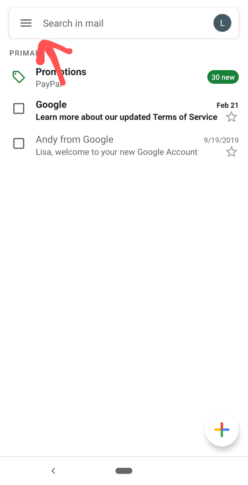The screenshot displays a mobile device's email interface, particularly showcasing how to use the 'Search in Mail' feature. Central to the image is a context menu with an option labeled 'Search in Mail,' highlighted prominently with a red arrow pointing towards it. On the far right of the search menu box, there's an oversized 'L,' likely representing a user icon. The interface also shows various email notifications: a green circle containing the number '30' indicates new promotions from PayPal, while another notification from Google about updated Terms of Service (dated February 21st) appears unchecked. Additionally, an older welcome email from Andy at Google, dated September 19, 2019, suggests the user hasn't reviewed their emails in several months. The bottom right corner of the screenshot features a multicolored plus symbol, alongside home and back buttons, confirming the mobile origin of the screenshot. Overall, the image serves as an informative guide on searching through mail on a mobile device.